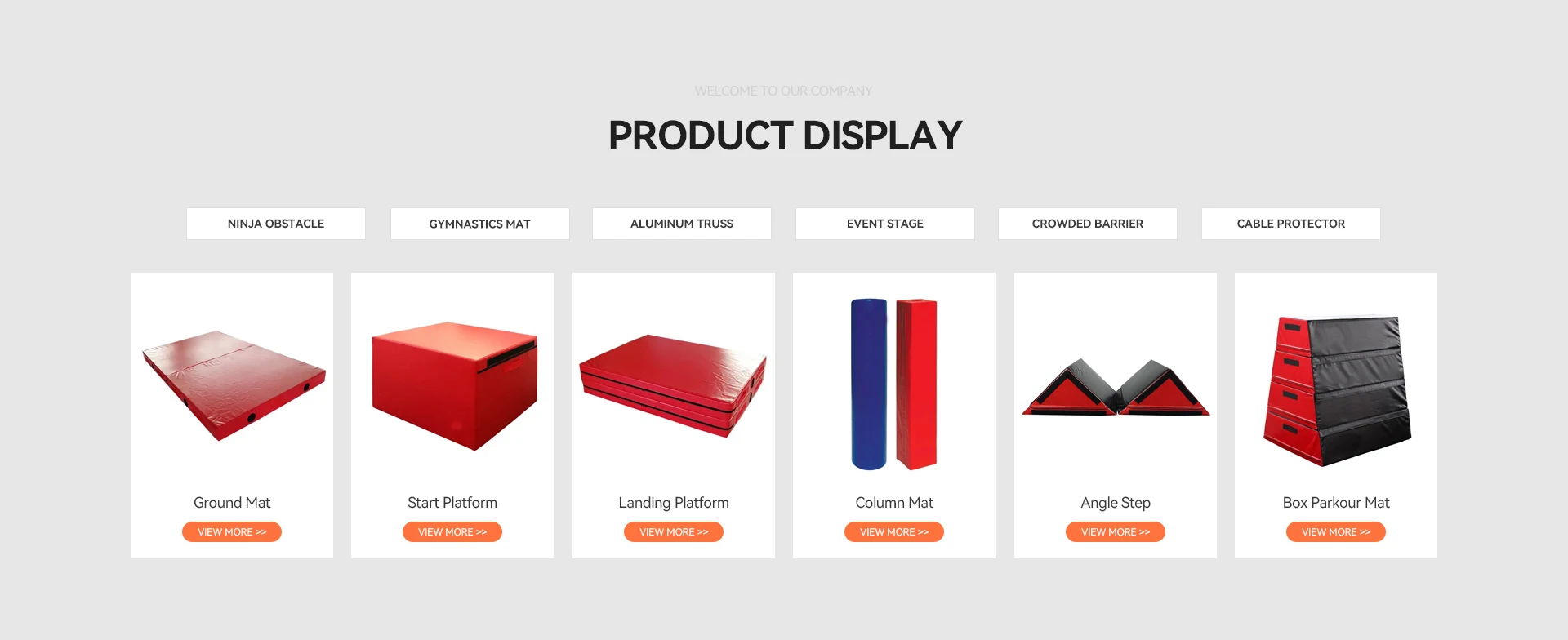The image is a long, rectangular layout with a light gray background at the top. At the very top, there is a faint gray text that reads "Welcome to Our Company." Below this, in large, capitalized black letters, the text "PRODUCT DISPLAY" appears. This top section of text is neat and justified, meaning all the lines are the same length.

At the bottom of the image, there are several rectangular menu options with white backgrounds and light gray borders. The menu options are listed in small, capitalized black font. The first menu option reads "NINJA OBSTACLE," followed by "GYMNASTICS MAT," "ALUMINUM TRUSS," "EVENT STAGE," "CROWD BARRIER," and "CABLE PROTECTOR."

Directly below these menu options are long rectangular images, each with a white background. Each image features a product with a black text label and an orange oval icon that is clickable, marked with "VIEW MORE" in white font along with double arrowheads pointing to the right.

- The first image shows a ground mat with the "VIEW MORE" oval icon at the bottom.
- The second image showcases a starting platform.
- The third image presents a landing platform.
- The fourth image displays a column mat, with one option in dark blue and oval-shaped on the left, and another in red and square-shaped on the right.
- The fifth image highlights an angle step, represented as two triangles with a red base and black border.
- The last image features a box parkour mat, consisting of several cylindrical shapes stacked together to form a giant rectangle. The sides of these shapes are black, while the fronts are red, each with a black handle in the center.